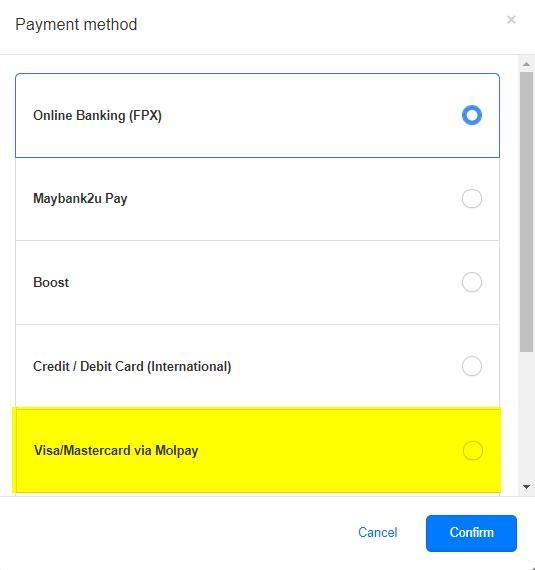The image is a screenshot of a payment method options window. At the very top left corner, it is labeled "Payment Method," with a small 'X' icon on the right side, providing a way to close the window. There are several payment options listed vertically. The first option, "Online Banking (FPX)," has a blue filled circle to its right indicating it is the currently selected option. The subsequent options are "Maybank 2U Pay," "Boost," and "Credit/Debit Card (International)." The final option, "Visa/MasterCard via MallPay," stands out as it is highlighted with a neon yellow marker color, indicating emphasis or possible selection.